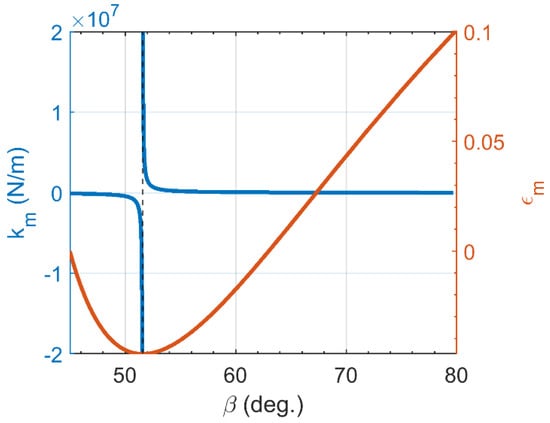This image features a detailed graph predominantly in blue and orange tones with some black accents. The vertical axis on the left, labeled in blue as KMN-M, displays values ranging from -2 to 2, with an exponent notation in the top left corner indicating times 10 to the 7th power. The horizontal axis, marked in black, spans from 50 to 80 representing BDEG, with SI units in degrees. On the right side, an orange vertical axis labeled 'E' shows values of 0, 0.05, and 0.1.

Within the graph, there are gray boxes scattered in the image. Two distinct blue lines can be observed: one starts at the top, descends towards the middle, and runs across the graph, while the other starts in the middle and slightly extends past the 50-mark. Additionally, an orange line starts above the -1 mark, dips down, and then rises sharply up to the top corner at the 0.1 mark.